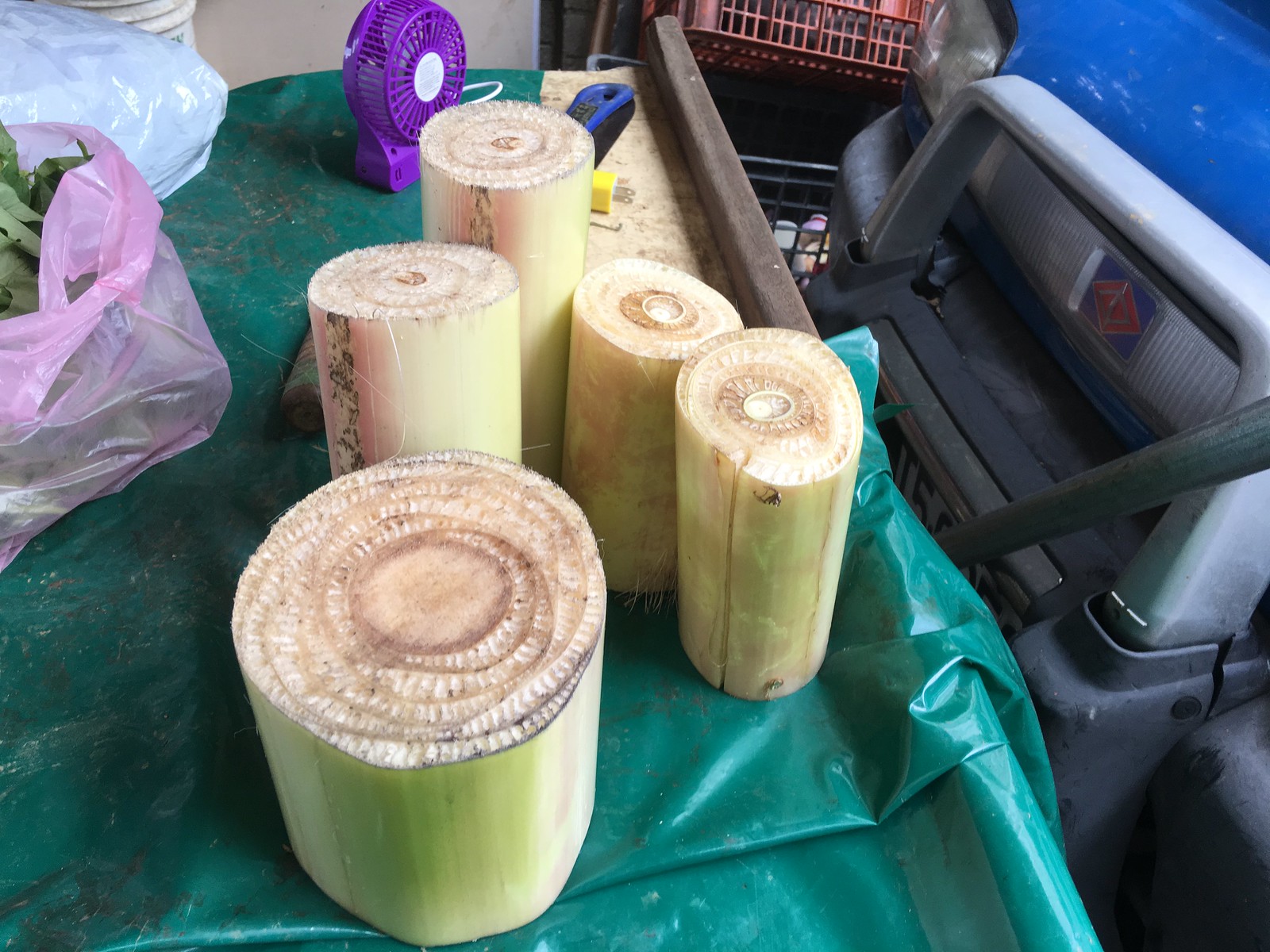The image depicts a scene in a garage or workshop area, where a green tarp covers a table or shelf. On the tarp, there are five cylindrical objects that resemble slices of large, light green and white gourds or bamboo, cut in a tapered manner akin to candles. Their interiors exhibit a cream and tan color with distinct rings, looking like dried loofah sponges or possibly sugarcane or other fibrous plant material.

Positioned towards the upper left of the frame is a small, purple desk fan angled to the right. To the left of these cylindrical objects, there is a pink plastic bag containing greenery, possibly lettuce, and another white bag with obscured contents. In the background, somewhat to the right, there is a compact vehicle, like a small truck or forklift, with only its front end visible. Additionally, red plastic boxes can be seen in the center background, adding to the cluttered yet intriguing composition of the scene.